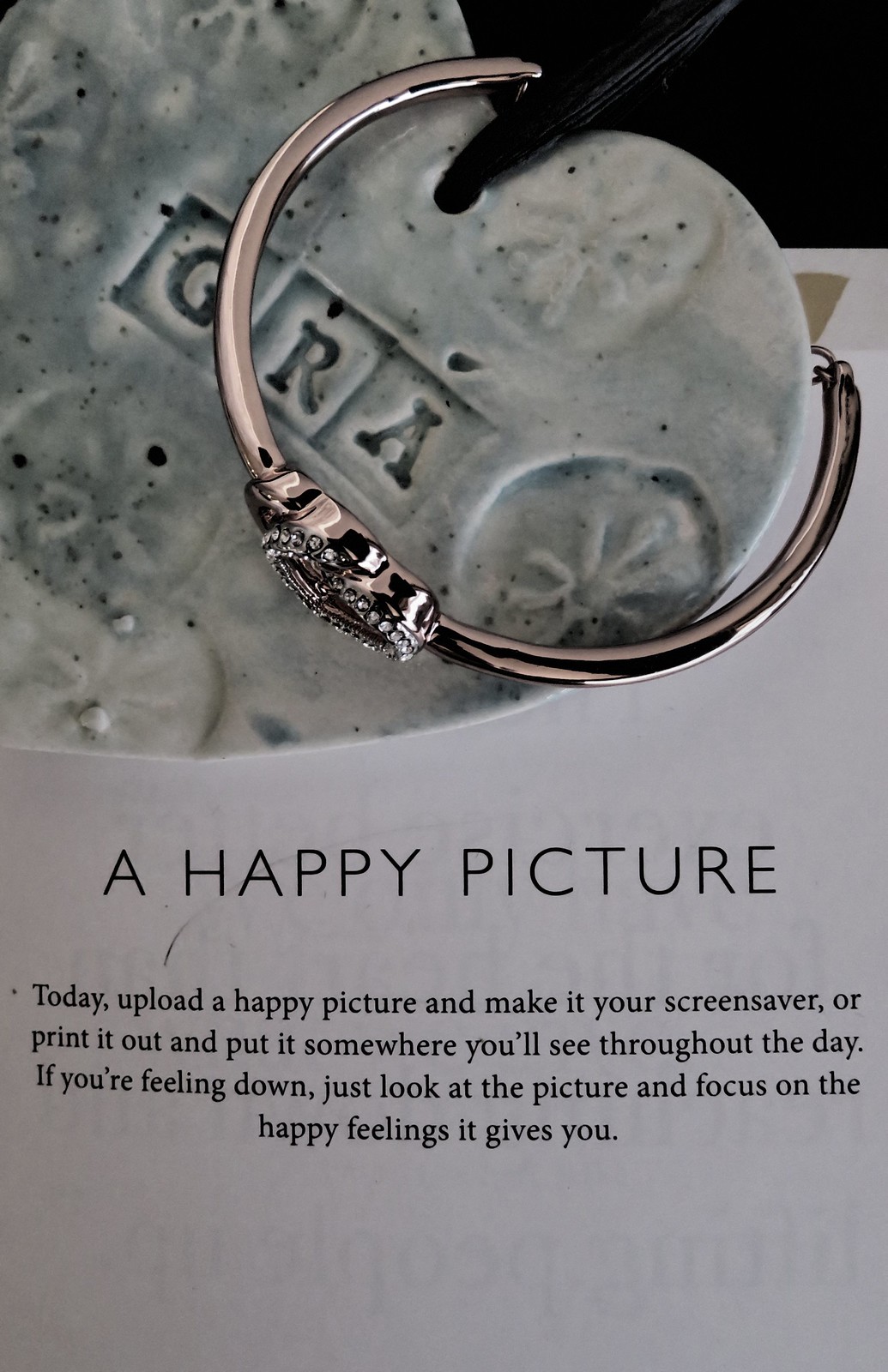The image showcases a silver piece of jewelry, likely a bracelet due to its curved shape and chain link connecting the two ends, elegantly wrapped around a stone heart. The heart, resembling a pendant, is primarily white with black markings and dotted imprints, and bears the engraved characters "G, R, A". Furthermore, it features a hole through which a string passes. Positioned at the bottom of the image is a black title in all capital letters stating "A HAPPY PICTURE", followed by a paragraph of smaller text. The paragraph encourages viewers to upload a happy picture and use it as a screensaver or print it out and place it somewhere visible throughout the day. It suggests that when feeling down, one should look at the picture and focus on the happy feelings it evokes.